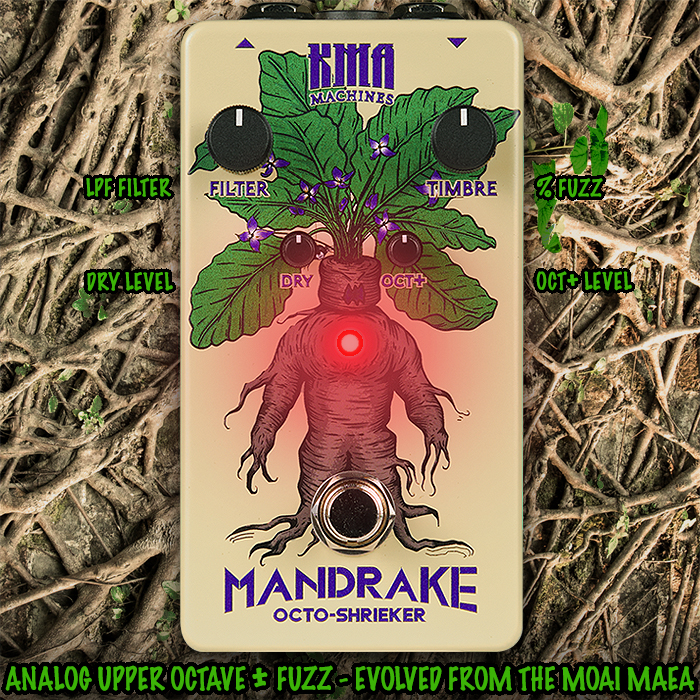This image features a detailed, hand-drawn advertisement for a product called the Mandrake Octoshrieker by KMA Machines. The object depicted is a tall, light beige rectangle with curved corners, set against a background of light brown tree roots interspersed with small leaves. At the top of this rectangular object, there are two black dials with white vertical lines at the top. The left dial is labeled "Filter" and the right one is labeled "Timbre." Below these are two smaller dials labeled "Dry" on the left and "Oct+" on the right.

The central image on this object is a cartoon-style anthropomorphized mandrake root with a head, arms, and legs, screaming with a red light in the center of its body; green leaves and small purple violets protrude from its head. The background features wooden textures and cord-like veins, giving it an organic and somewhat eerie appearance.

On the left side of the object, there is a label indicating an LPF filter, and on the right side, there is a notation about the percentage of fuzz. At the bottom of the image, "Mandrake Octoshrieker" is written in bold purple font, and beneath that, in green font with a black outline, it reads "analog upper octave" and "fuzz evolved from the Mau Mayo."